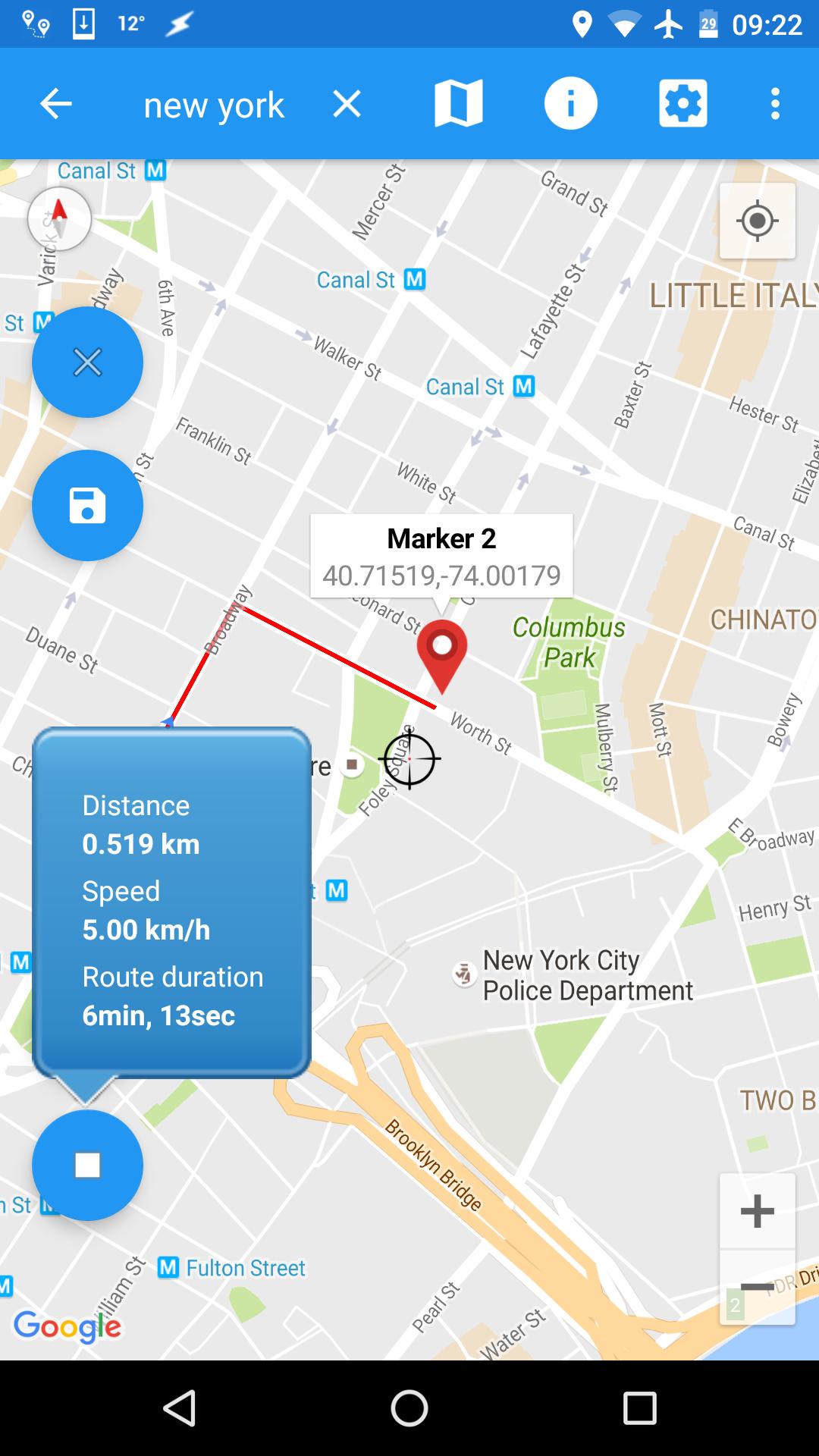The image depicts a navigation screen on an unspecified maps application focused on New York City. The map highlights a route beginning on Broadway, indicating a peculiar navigation instruction to travel the wrong way down a one-way street. Key landmarks visible include the New York City Police Department and the Brooklyn Bridge. The route commences near the intersection of Foley Square and Worth Street, marked for an unknown reason. The distance to the marker is 0.519 kilometers, with an estimated travel time of six minutes and 13 seconds at a speed of five kilometers per hour, suggesting typical heavy traffic for the area. The map interface is predominantly plain with a blue bar at the top providing additional options and filters.